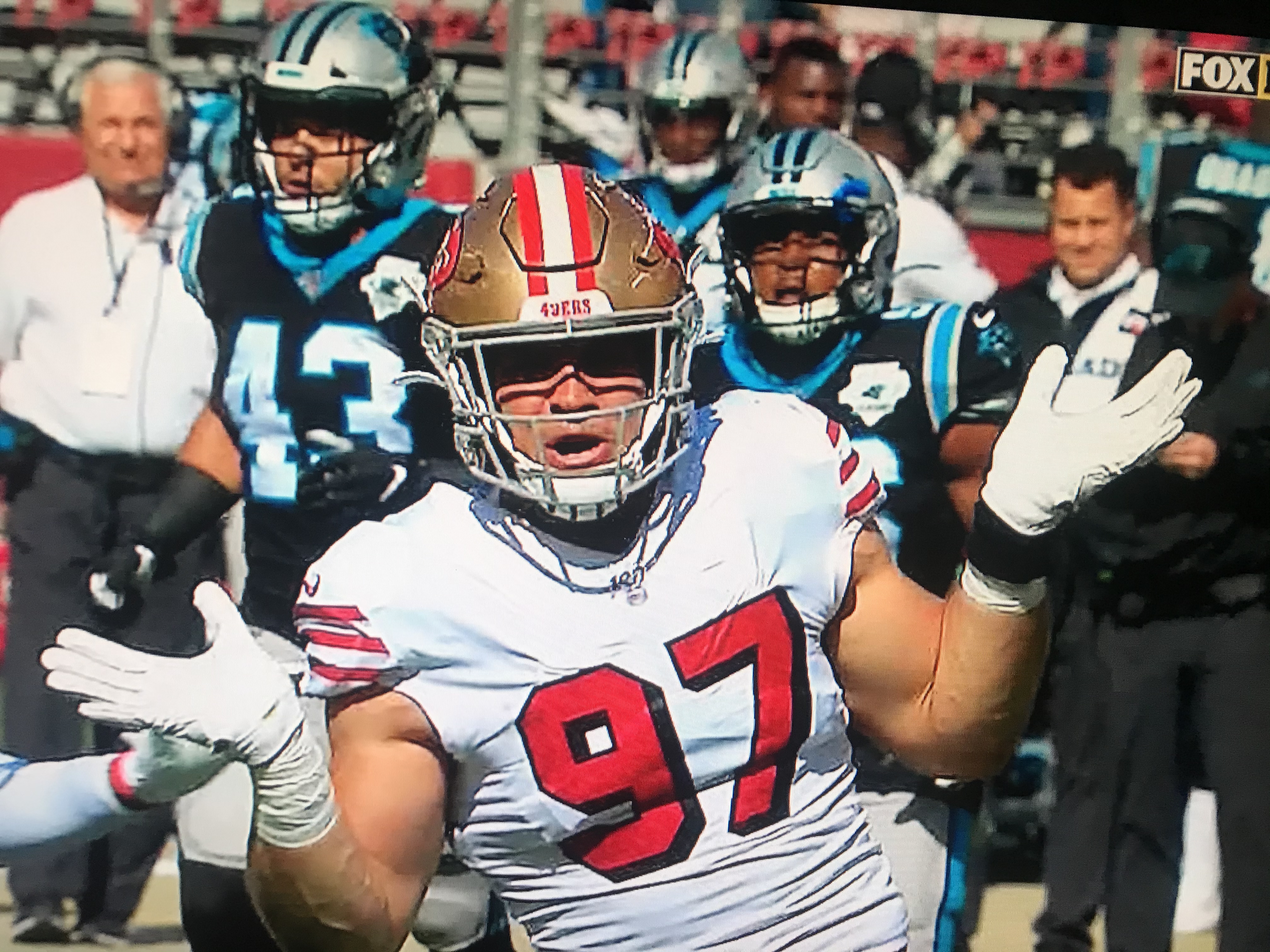This image captures a moment during a football game featuring a player from the 49ers prominently in the foreground. The player's gold helmet with "49ers" inscribed in white stands out, along with his white jersey marked by the red number 97 and three red stripes on each sleeve. He appears to be speaking or calling out, adding dynamic energy to the scene. His attire is further complemented by white gloves, emphasizing his readiness for action. 

Slightly out of focus behind him, a man gestures with both arms raised in an "I don't know" manner, possibly a coach or supporter expressing confusion or frustration. Additionally, three football players in dark blue or black jerseys with white numbers are visible; one, marked with the number 43 outlined in light blue, stands out. To the far left, a news broadcaster, identifiable by his white shirt, dark gray trousers, and white hair, wears a headset, possibly reporting the live action. The background to the right shows more individuals, not in uniform, adding to the bustling atmosphere. Above, in the right-hand corner, the Fox Network’s logo is visible in white letters on a black background, indicating the game's broadcast on the Fox channel. The overall color palette includes black, white, red, blue, gold, and hints of brown, capturing the vibrancy of the game day scene.